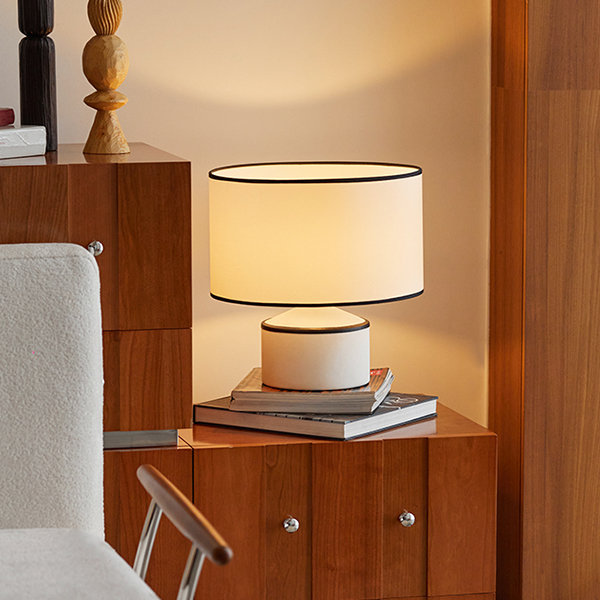The image depicts a modern, square walnut-colored nightstand or dresser with simple round chrome handles, creating a sleek and contemporary look. On its surface, there is a short and stout white table lamp with black rims on both the light and the shade, emanating a warm, yellow-tinged glow. The lamp sits atop a stack of books and magazines. To the left, a matching set of cabinets is visible, adorned with similar chrome handles. In front of the nightstand, there's a white Sherpa fabric chair with a chrome frame and walnut-tone wooden armrests. The overall ambiance suggests a cozy living room bathed in warm lighting, enhancing the inviting atmosphere.